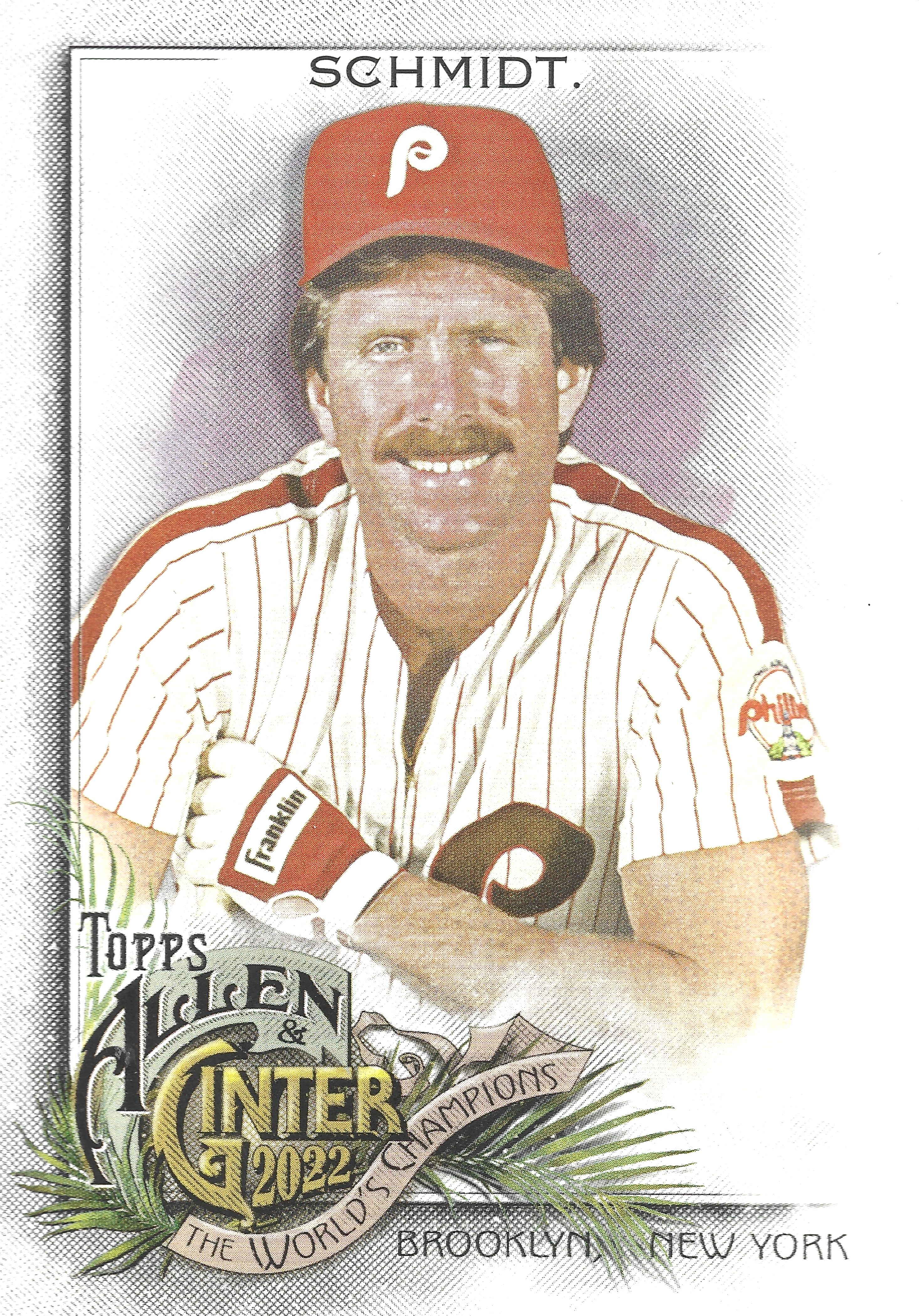The image is a detailed color illustration in portrait orientation depicting a notable baseball card from Topps Allen & Ginter 2022 series labeled "The World's Champions." The card prominently features Michael Jack Schmidt of the Philadelphia Phillies. Schmidt is shown smiling broadly at the viewer, sporting a red Phillies cap with a white "P" logo. His brown hair, mustache, and numerous freckles are clearly visible. Over his head, the name "SCHMIDT" is spelled out in all capital letters.

Schmidt is dressed in the Phillies' white jersey with thin red pinstripes and a thicker red stripe over the shoulders. The "P" emblem is partially visible on the left chest, and the jersey features a Phillies logo patch on the shoulder. He wears a white batting glove with a red band, prominently displaying the brand "Franklin" in black lettering on it. His arms are folded across his chest, partially covering the "P" logo.

At the bottom left corner of the card, there is the distinct Topps logo alongside the Allen & Ginter 2022 branding. Below it, a beige banner with black text states "The World’s Champions," and further down in black text is "Brooklyn, New York." The background features subtle artistic elements, including a green palm frond, blending photographic realism with graphic design.